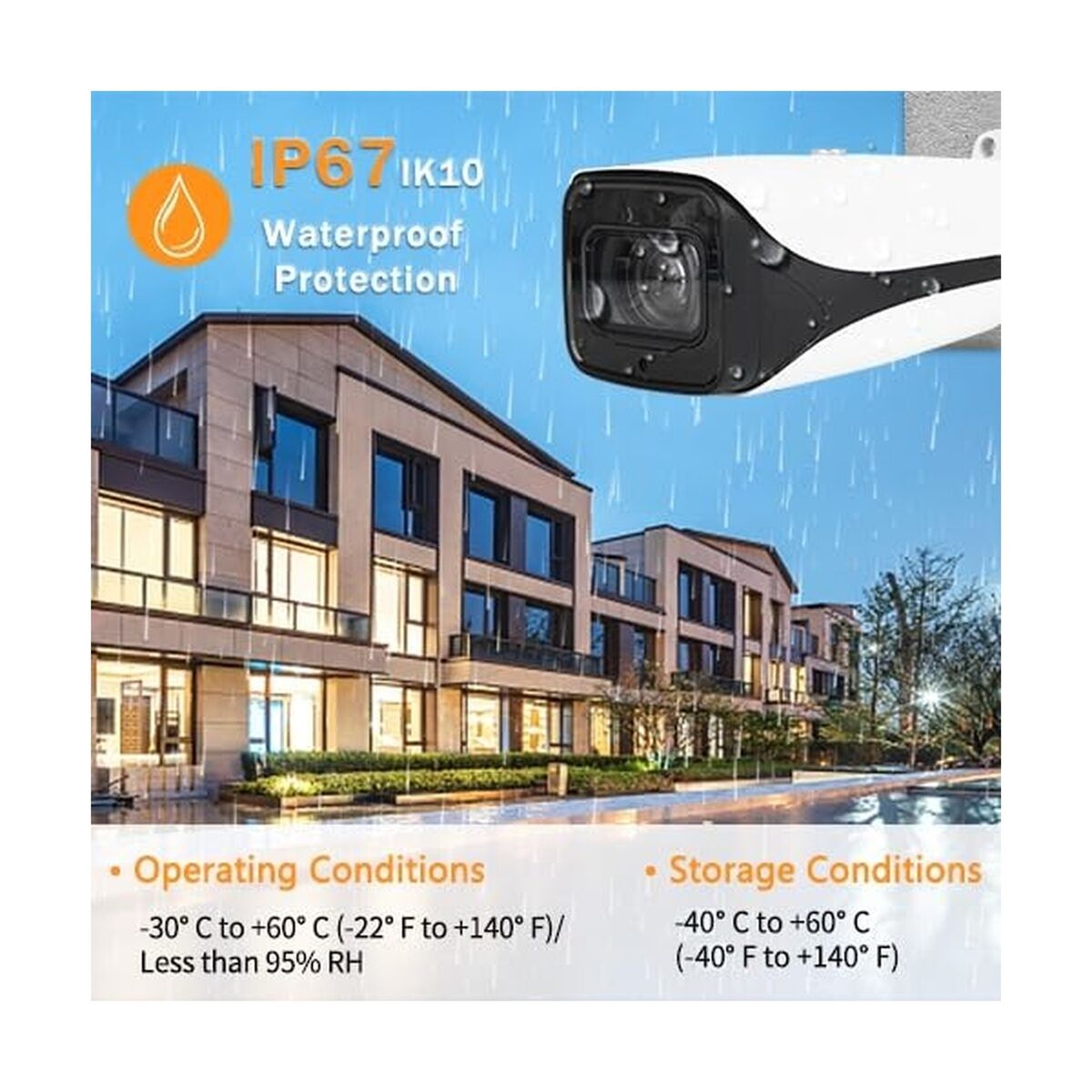The advertisement showcases an outdoor security camera with a sleek, white body featuring black accents, strategically positioned in the upper right corner of the image. The camera's waterproof capability is emphasized through visible water droplets on its surface and falling in the background, suggesting protection against harsh weather conditions, supported by the IP67 and IK10 waterproof protection rating prominently displayed in an orange color with a matching raindrop icon on the top left. The backdrop of the ad is a large, multi-story office building characterized by numerous glass windows, some illuminated, indicating occupancy. The building is surrounded by bushes and features a swimming pool edge visible on the lower right. On the bottom of the ad, information about the camera's robust performance in extreme temperatures is provided, detailing operating conditions from -30°C to 60°C (-22°F to 140°F) and storage conditions from -40°C to 60°C (-40°F to 140°F). The entire scene, from the architectural elements to the weather effects, underscores the camera's suitability for various environments.